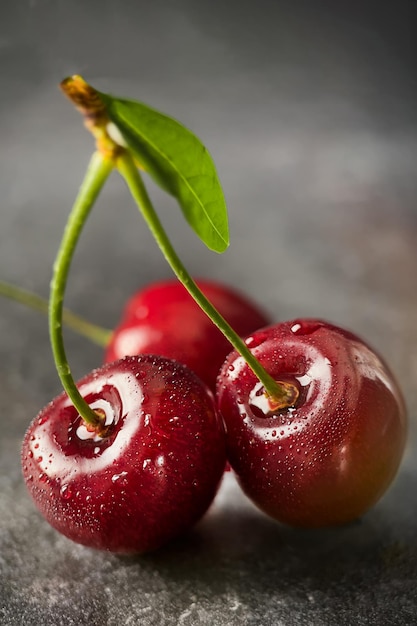A close-up photograph features three ripe cherries on a gray countertop that appears to be made of a material like Formica or granite. The countertop is gray with white flecks and the background transitions through different shades of gray, creating a soft, blurred effect. Two of the cherries are prominently displayed in the foreground, connected by their green stalks, with a tiny, lonely green leaf hanging from the tip. The third cherry is blurred in the background, lying on its side. The cherries are covered in dew, with droplets of water glistening on their deep red surfaces, reflecting light and accentuating their freshness and shine. This well-composed and aesthetically pleasing photograph captures the vivid contrast between the rich red of the cherries and the muted gray background, highlighting the cherries as the central focus.